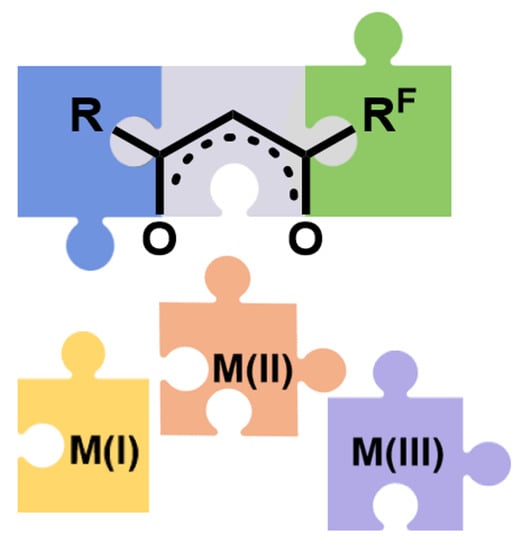The image features a series of six detailed puzzle pieces that seem to represent some form of molecular or chemical bond. At the top of the image, three puzzle pieces are connected in a row. The left piece is blue with a black letter 'R' on it, the middle piece is grey with a house shape or network of solid and dotted lines and possibly 'zeros', and the right piece is green with the notation 'RF' on it. Below this row, there are three additional puzzle pieces that are not connected to each other. The left piece is yellow with the characters 'M(I)', the middle piece is peach-colored with 'M(II)', and the right piece is a pastel purple with 'M(III)'. The overall arrangement and notations suggest these pieces might correlate to a molecular structure or chemical bonding pattern.